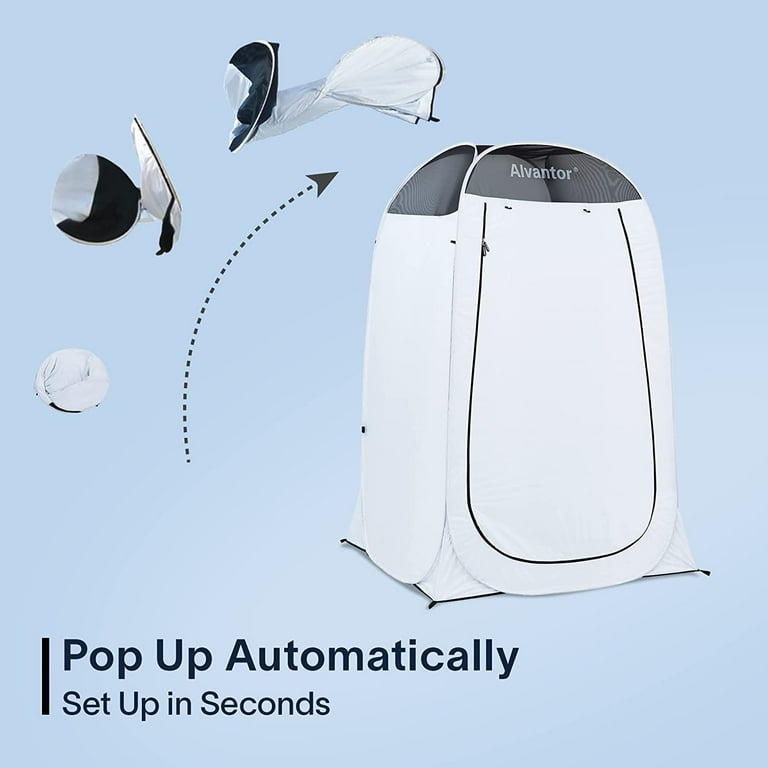This advertisement features a pop-up tent from the brand "Alvantor." The background is a light cyan color with a black line at the bottom, over which dark blue text reads: "Pop up automatically, set up in seconds." The main image displays the tent fully set up, which is predominantly white with a black top and black outlining the zipper. The brand name "Alvantor," styled in gray, is visible on the black vent at the top. On the left side of the advertisement, a sequence of images accompanied by a black arrow illustrates the tent's transformation from its packed state to being fully opened. This setup process emphasizes the tent's ease of use and quick assembly.